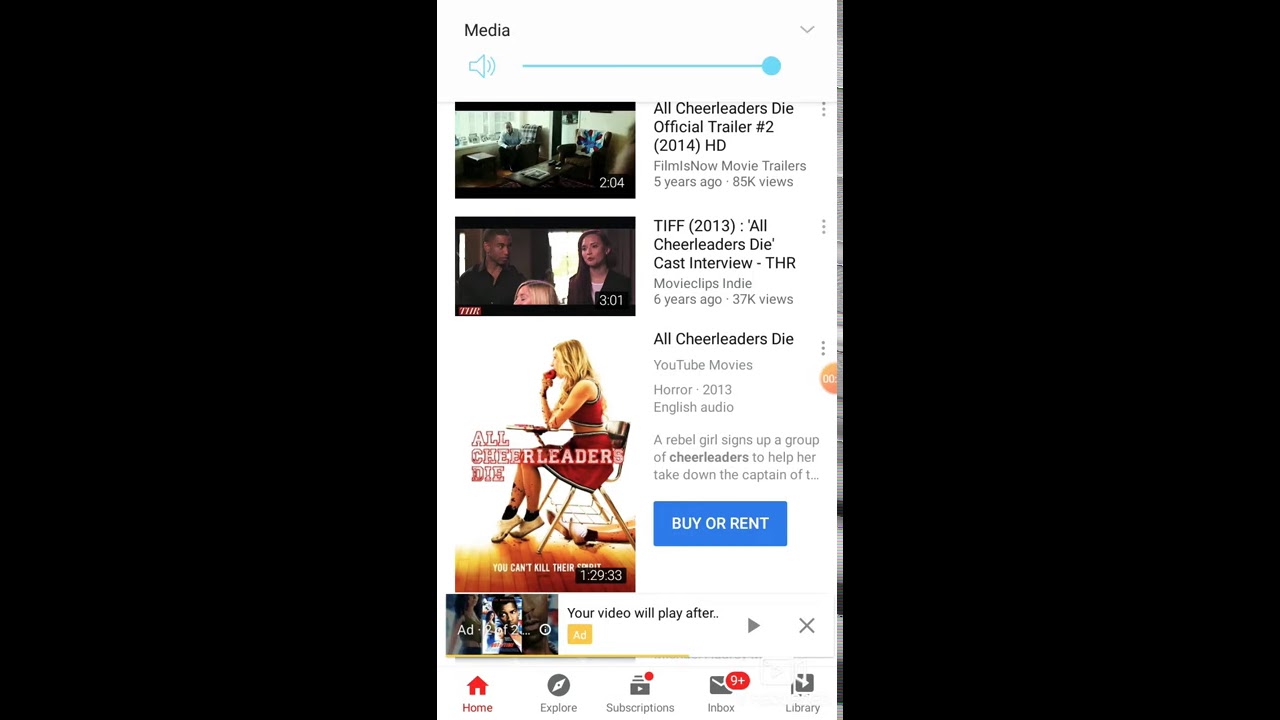In the center of the image, there is a long rectangular section containing various pieces of information. At the top of this section, the word "Media" is prominently displayed, accompanied by a blue speaker icon with three short lines emanating from it, indicating sound.

To the right of this, there is a light blue horizontal line with a blue circle at one end. Below this main section, there are multiple video options listed:

1. The first video option features a clickable thumbnail showing a man sitting in a living room. The video's duration is indicated as 2:04. To the right of this thumbnail, the text reads "All Cheerleaders Die, Official Trailer #2 (2014) HD".

2. The second video option has an image of a woman and a man in a black shirt sitting in a room. The video's duration is 3:01. To the right, the text reads "TIFF (2013) All Cheerleaders Die Cast Interview".

3. The third section displays the front cover of the movie "All Cheerleaders Die", showing a girl in a red cheerleader uniform sitting at a school desk. To the right, it reads "All Cheerleaders Die, YouTube Movies, Horror, 2013, English Audio" alongside options in a blue box to "Buy" or "Rent" the movie. The runtime for this movie is displayed as 1 hour 29 minutes.

At the bottom of this detailed informational rectangle, there is a note stating that the video will play after an ad.